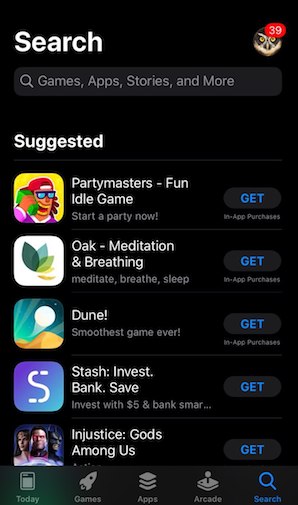The image captured from a cell phone screen showcases a search interface against a black background. At the top of the screen, "Search" is displayed in white font, followed by a search bar containing a magnifying glass icon. Inside the search bar, the placeholder text reads "games, apps, stories, and more" in gray.

Below this, on the left side, the section titled "Suggested" features a list of five apps or games. The first app, "Party Masters," is described as a "fun idle game" and is accompanied by a blue "Get" button on the right. The app's icon depicts a man holding a green object near his head.

The second app is "Oak: Meditation and Breathing," represented by a white square with green leaves in its icon. It also has a blue "Get" button on the right side.

Next is an app with the title "Dune," identifiable by an icon with teal and tan colors and a white bar. This app similarly includes a blue "Get" button.

The fourth app, named "Stash: Invest, Bank, and Save," features a blue square icon with a white 'S.' The "Get" button remains consistently blue.

Lastly, the app "Injustice: Gods Among Us" is listed but lacks additional descriptive elements or icon details in the provided text.